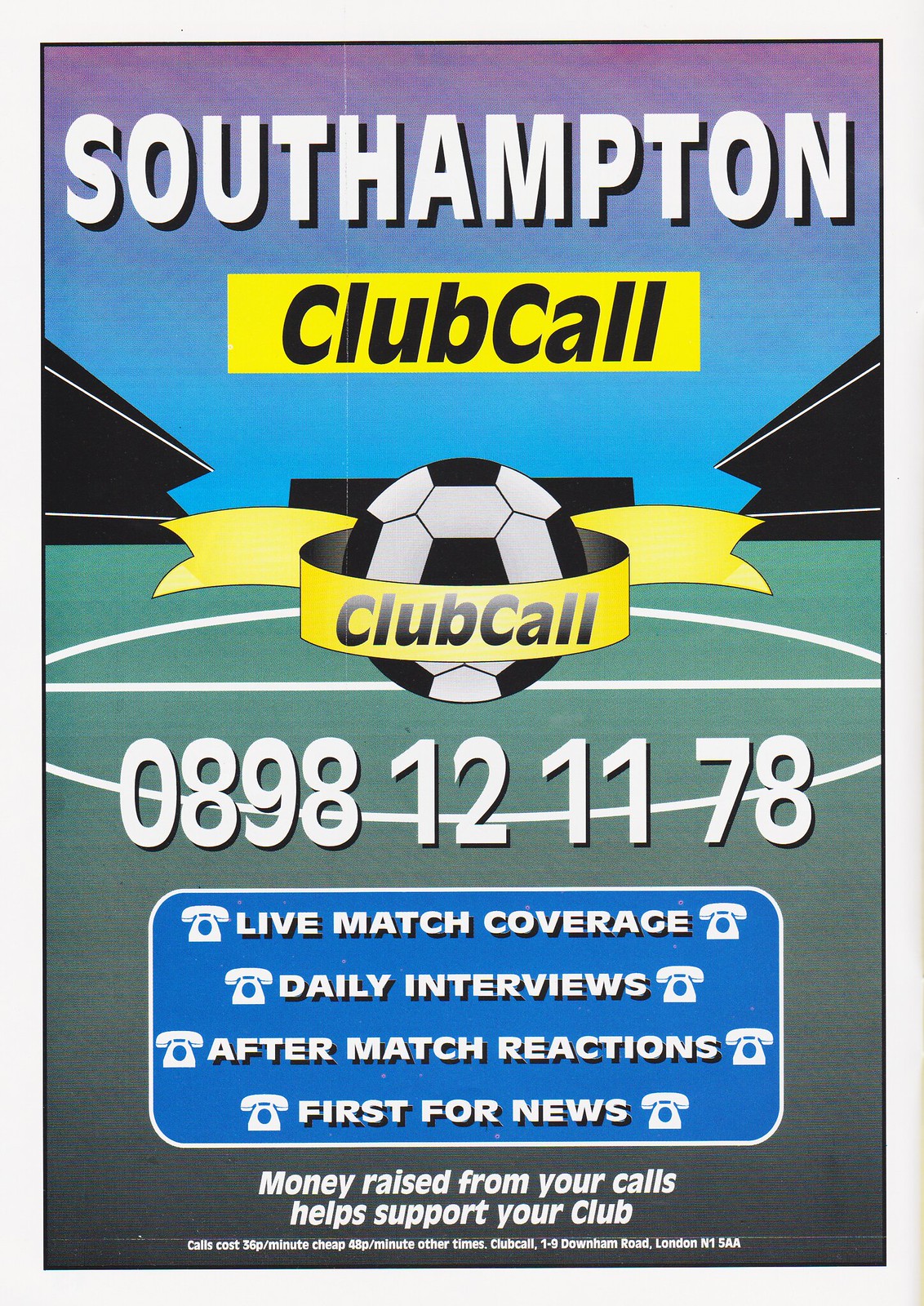This is an advertisement for Southampton Club Call encouraging supporters to make calls to support their club. The image prominently features a digitally-rendered soccer field with a floating soccer ball wrapped in a yellow ribbon that reads “Club Call” at the center. Surrounding the ball, the text reads: "Southampton Club Call 0898-12-1178." Additional features include animated elements like bleachers and white painted lines on the field, enhancing the visual appeal. A blue box on the poster lists services provided: "Live match coverage, Daily interviews, After match reactions, First for news." Below this, smaller text states, "Money raised from your calls helps support your club. Calls cost 36p per minute and 48p per minute at other times." Lastly, the poster includes the address, "Club Call, 19 Down Road, London, N15 8."